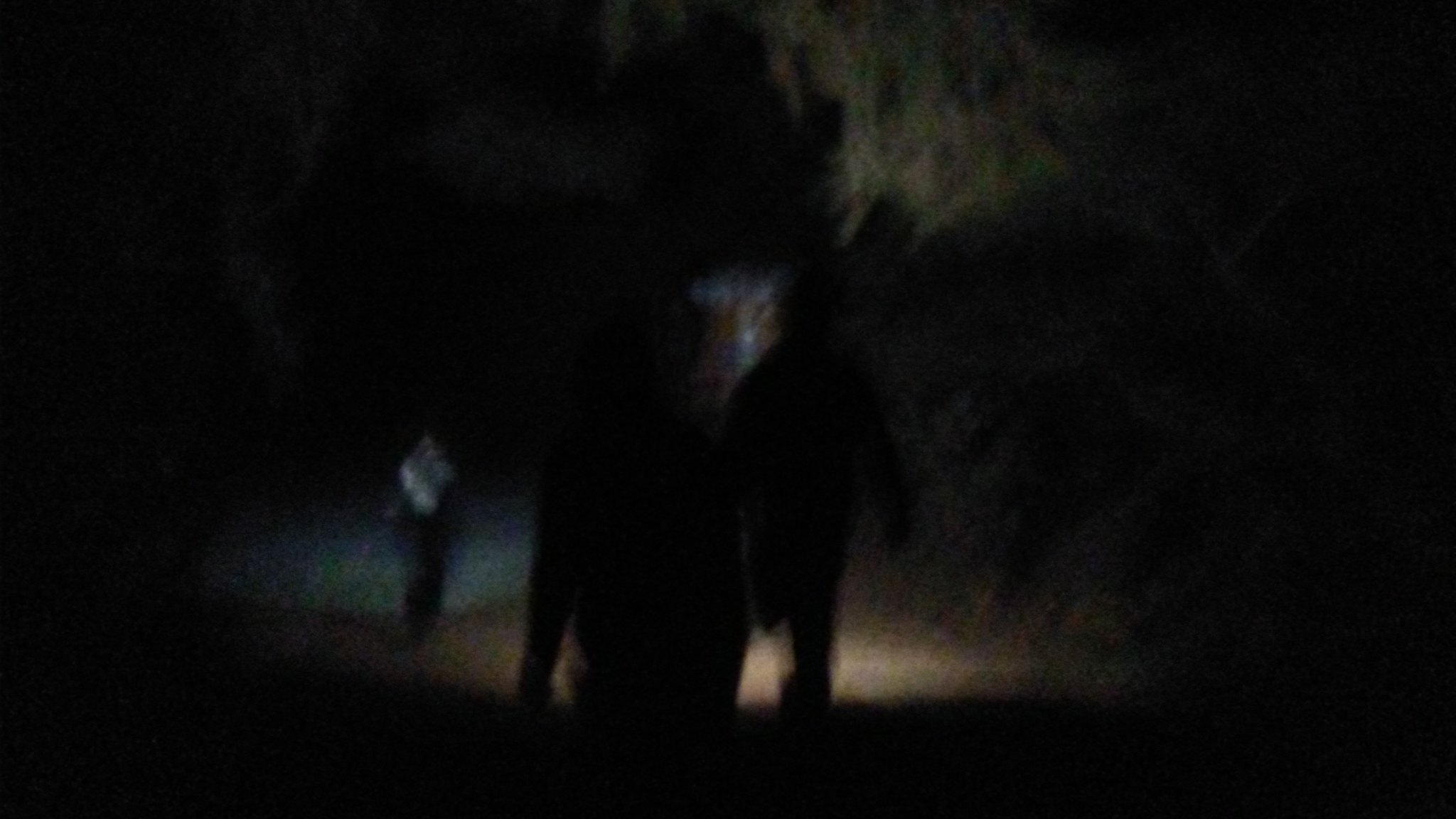This is a very dark and blurry photograph, likely taken outside in the middle of the night. The image is horizontally-oriented and depicts an eerie scene reminiscent of a scary movie. In the center, there appears to be a menacing figure with arms hanging at its sides. Its face is a blur of brown, green, purple, and white, giving it an almost ectoplasmic appearance. Behind this central figure, to the left, stands another dark figure, slightly illuminated around the torso and head, possibly creating shadows. The ground in front of the rear figure is illuminated, perhaps by a headlamp or flashlight. The overall scene is bathed in darkness with minimal light, revealing sparse details like a little brown on the ground and dark green trees towards the right of the image.